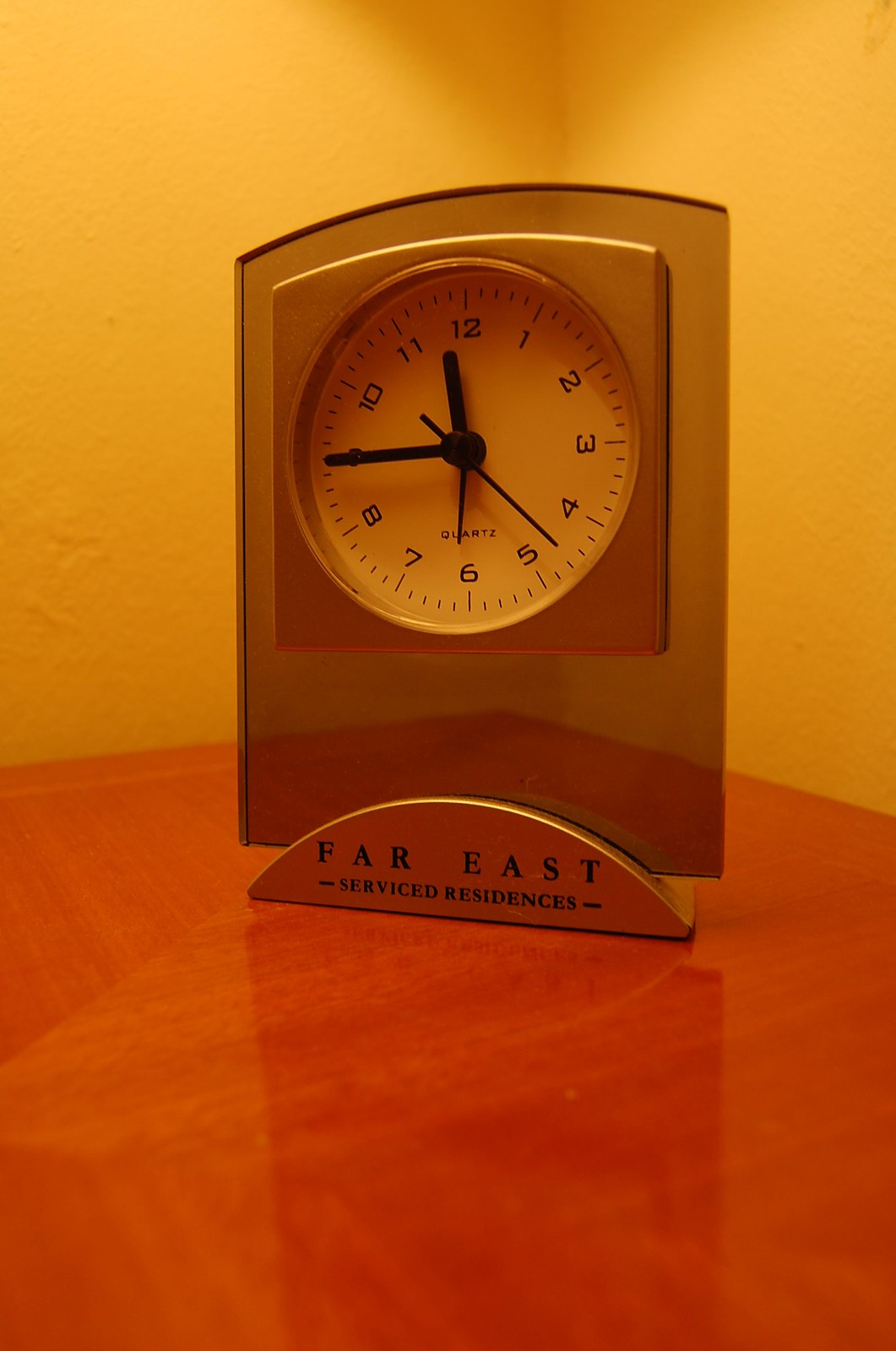A polished, reddish wooden desk serves as the elegant base for a sophisticated desk clock in this photograph. The clock, marked "Far East Service Residences" at the bottom, sits firmly on its half-circle base. The timepiece itself features a slightly curved rectangular frame, accentuating its modern design. The pristine white clock face is adorned with three sleek black hands – an hour hand, a minute hand, and a second hand. The time is captured at 11:45, with the small hour hand positioned slightly closer to 12 and the larger minute hand pointed directly at 9. The backdrop reveals a cozy room with warm, tan-yellow walls, enhancing the overall inviting ambiance of the scene.